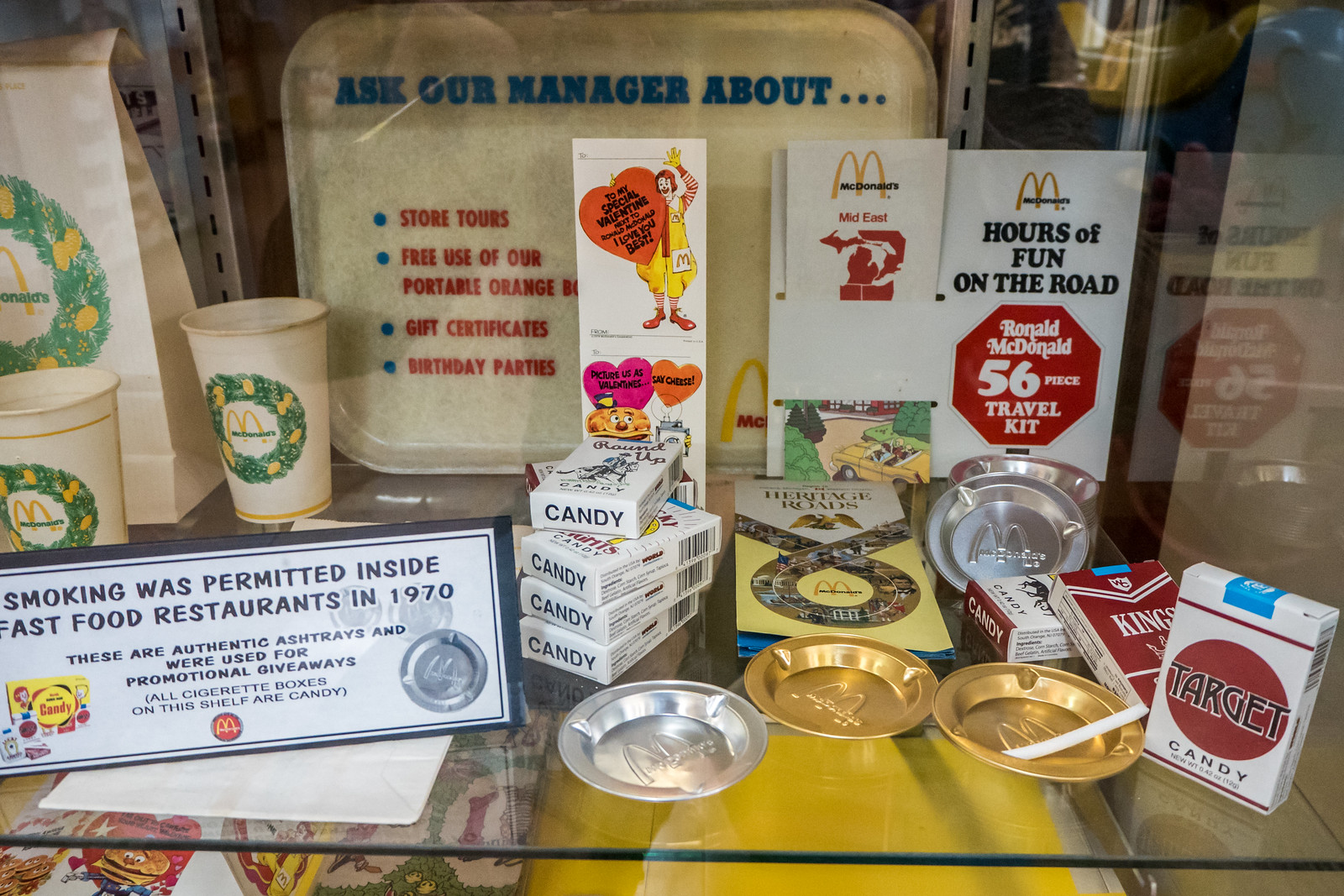This image depicts a meticulous display case indoors, seemingly part of a McDonald's museum exhibit or a collection of McDonald's memorabilia. The central focus is a glass shelf holding an assortment of vintage items scattered across its surface. Prominently featured are authentic gold and silver ashtrays, once used for promotional giveaways when smoking was permitted inside fast food restaurants in 1970, alongside white and red boxes clearly marked as candy cigarettes. Surrounding these are various McDonald’s artifacts, including travel pamphlets like "McDonald's Mideast" and "McDonald's Hours of Fun on the Road," a 56-piece Ronald McDonald travel kit, McDonald’s cups, bags, and posters. The colors in the image range from yellow and gold to silver, red, blue, green, gray, and tan, enhancing the nostalgic ambiance of the exhibit. An informative sign at the bottom left reads, "Smoking was permitted inside fast food restaurants in 1970," underscoring the historical context of the displayed items. For added interactivity, there's an invitation to ask the manager about store tours for the use of portable orange gift certificates for birthday parties.